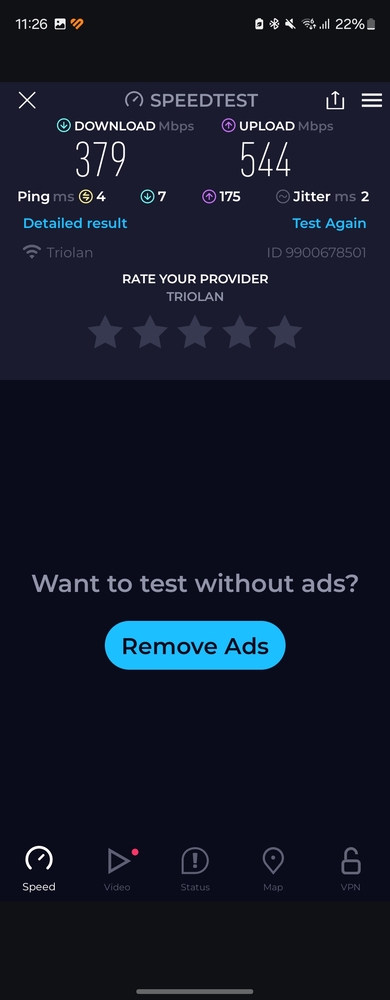This image is a detailed screenshot of a speed test application interface. 

In the top left corner, there are various cell phone icons followed by the time "11:26," a gallery icon, and an orange icon. On the right side, additional cell phone icons are present, with a battery percentage indicator prominently displaying "22%." The background of this top section is black.

The main portion of the screen, set against a gray background, prominently displays "Speed Test" with metrics for "Download MBPS" and "Upload MBPS," indicating it measures internet connection speeds. Below these metrics, details such as "Ping MS" showing a value of 7, a reading of 175 next to "Jitter MS," and two blue options, "Test Again" and "Detailed Result," are visible. A Wi-Fi icon is also present, indicating the test is being conducted on a Wi-Fi network provided by "Triolin."

Further down, the interface encourages users to "Rate Your Provider, Triolin," out of five stars. There is also a promotional message asking, "Want to Test Without Ads?" followed by a turquoise oval button with "Remove Ads" written in black text inside it.

At the bottom of the screen, there are five navigational icons: "Speed," "Video," "Status," "Map," and "VPN," all set against another black background.